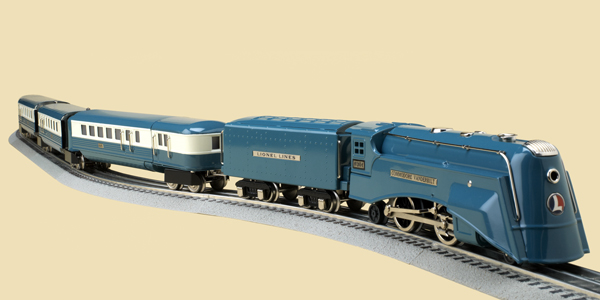The close-up image features a meticulously detailed model train set against a flat beige background. The train, which runs diagonally from approximately the left side of the image to the bottom right-hand corner, appears almost old-fashioned, reminiscent of tin train models. The track is rendered in black and gray, with gray pebbly shapes flanking its sides, giving the illusion that it continues beyond the frame. The train comprises five cars: the engine and four passenger cars. The first two units, the engine and a linked car, are painted in a dark royal blue and bear the emblem "Lionel Lines" prominently on their sides. Following these, the three passenger cars showcase a royal blue paint scheme accented by a creamy stripe running through the middle where rectangular windows are positioned, providing a classic look. The train sits fully on its track, encapsulating the nostalgic charm of vintage railway models.